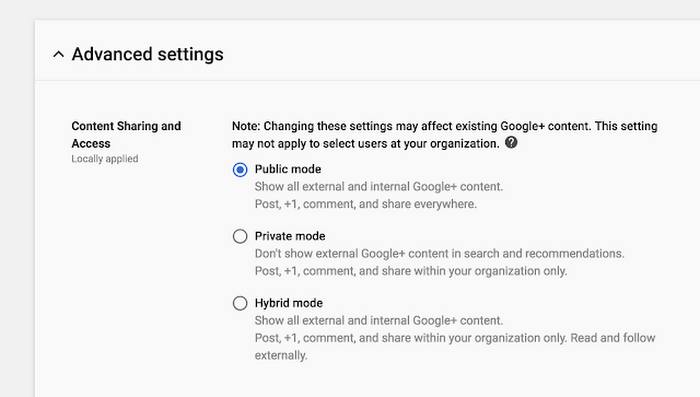Screenshot of a computer screen displaying a user interface with a light gray background and a slightly lighter gray rectangle in the foreground. At the top of this interface, the text "Advanced Settings" appears in black, accompanied by an upward-pointing arrow on the left side. Below this title, the text "Content Sharing and Access" is displayed, followed by the phrase "Locally applied."

In the central portion of the interface, a black text note reads, "Note: Changing these settings may affect existing Google Plus content. This setting may not apply to select users at your organization," ending with a question mark.

Three selectable options with circular toggle buttons are visible, each with descriptive text:
1. **Public Mode**: A blue circle indicates that this mode is currently selected. The accompanying description states, "Show all external and internal Google Plus content. Post, +1, comment, and share everywhere."
2. **Private Mode**: Describes limiting the visibility to internal content only, with the text, "Don't show external Google Plus content in search and recommendations. Post, +1, comment, and share with your organization only."
3. **Hybrid Mode**: Positioned below the other options but lacks a detailed description in the provided text.